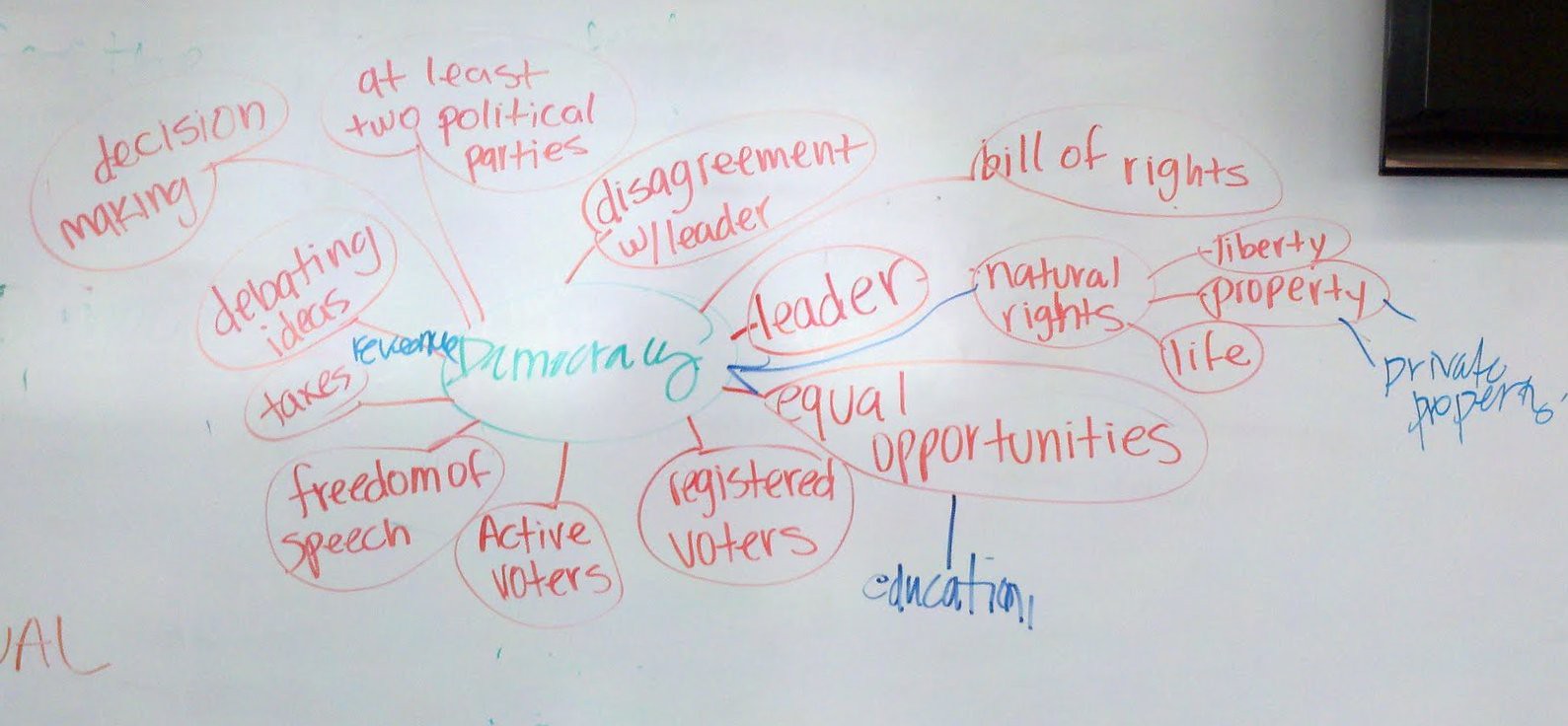The image depicts a whiteboard in landscape orientation, covered with a detailed bubble chart written in colored markers. At the center of the chart, the word "democracy" is highlighted in green. Emanating from this central word are numerous red lines, each connecting to red-circled ideas that collectively outline key components of a democratic system. These include decision-making, debating ideas, taxes, freedom of speech, active voters, registered voters, equal opportunities, leaders, disagreement with leaders, at least two political parties, and education. In addition to red, some blue lines and circles further elaborate on certain concepts such as private property and education. To the right, the fundamental principles of natural rights, liberty, property, life, and the Bill of Rights are also included. The photo is well-organized with clear, legible handwriting and resembles notes from a government or civics class, providing a comprehensive depiction of the elements that constitute democracy. In the top right corner, a black speaker is partially visible, adding a subtle context to the indoor scene.